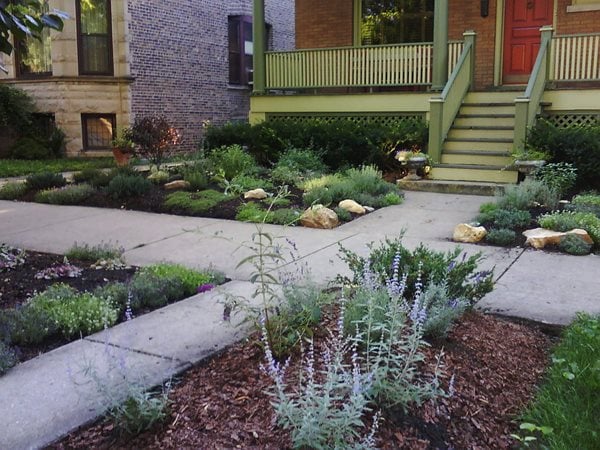This color photograph, taken in landscape orientation from the street, showcases the newly landscaped front yard of a red brick house with a red door. The image captures a concrete walkway that intersects with a public sidewalk and leads to a staircase ascending to the porch. The staircase is painted green with darker green hand railings, complemented by yellow railings at the top. The front yard features fresh mulch and an array of new plants, including bright green shrubbery with small white flowers, light mint-colored plants with small purple flowers, and a noteworthy reddish-colored shrub. Speckled among the mulch are light brown rocks. Beneath the porch is neatly installed lattice work. To the left of the house, there is a large brick building with a lighter façade and numerous windows, adding to the urban residential scene. Small patches of grass are visible on the bottom right and side of the walkway, enhancing the garden-like quality of the yard.